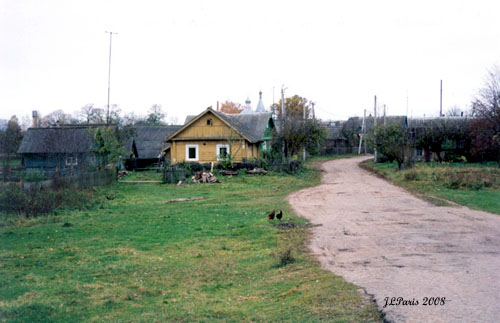This photograph captures a quaint scene centered around a small, mustard-yellow house with a dark gray rooftop. The house is situated in a lush green grass area, which is lush and expansive. Surrounding this house are several other buildings, all sharing the same dark gray rooftops, indicating a visually cohesive neighborhood. The photograph also features a winding beige pathway, surrounded by green grass, leading toward the back of the image. This pathway is flanked by signs of animal life, notably two chickens strolling in the grass.

On the left side of the photograph, there is a driveway or a road that stretches across the green area. The road appears grayish-white with hints of black, and at the bottom right corner, there is an inscription that reads "JL Paris 2008," partially cut off from the image. Alongside the road, there are white posts standing upright, creating a sense of symmetry. The road and pathway intersect the grass, which shows patches of brown dirt and areas with green bushes and trees, some of which have reddish leaves.

To the left side of the mustard-yellow house, a series of housing units is visible. The first of these is a blue house with a black roof, followed by another yellow house with a similar black roof. Next is a green house, also topped with a black roof, showcasing a neighborhood with a harmonious color theme. The sky above is white, casting a soft, diffused light over the scene.